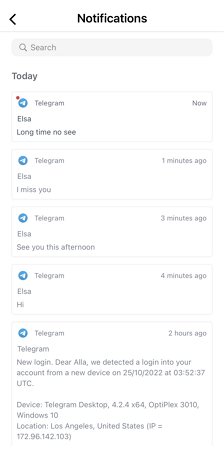In this vertical screenshot, likely taken from a smartphone device, the primary focus is on a series of notifications. The top portion of the image displays the header "Notifications" in bold, black text, centrally aligned. To the left of the header, there is a small left-pointing arrow. Below this section, a light gray line acts as a separator. 

Directly beneath the separator is a search bar, marked with a magnifying glass icon, allowing the user to search through their notifications.

Underneath the search bar, the bold text "Today" signifies the start of the day's notifications. The following notifications, all from the messaging app Telegram, are listed in descending chronological order. The first notification from Telegram reads, "Elsa, long time no see," followed by "Elsa, I miss you," received one minute ago. Another notification from Elsa states, "See you this afternoon," received three minutes ago, and finally, "Hi," received four minutes ago.

Further down, there is a more detailed notification regarding a security alert. This message from Telegram indicates a new login attempt: "New login: Dear [User], we detected a login to your account from a new device on 25/10/2022 at 3:52:37 UTC." This section also includes detailed device information and shows the location as Los Angeles, United States, with the IP address 1.72.96.142.103, dated two hours ago.